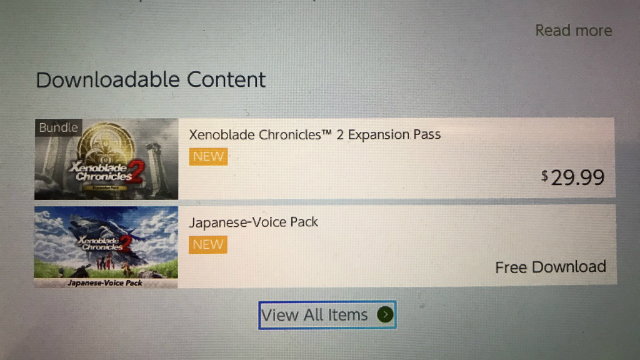This photograph captures a TV or computer screen displaying downloadable content for a video game. The screen features a faint line pattern, indicative of the image being taken with a camera. The top left corner prominently displays the words "Downloadable Content" in large black font. Below this heading, there are two elongated white rectangles, each containing a game thumbnail on the left, followed by the game title on the right.

The first rectangle shows the thumbnail for "Xenoblade Chronicles 2 Expansion Pass." Directly to the right of this thumbnail is the game title, and underneath it, a yellow box with the word "New" in large white letters. To the far right of this box, the price is listed as "$29.99."

The second rectangle features the thumbnail for the "Japanese Voice Pack for Xenoblade Chronicles 2." Similar to the first listing, the game title is positioned to the right of the thumbnail, with a yellow box indicating "New" beneath it. To the right, it states "Free Download." 

At the bottom of the screen, the phrase "View items" is displayed, highlighted in a blue box, suggesting users click to see all available downloadable content.